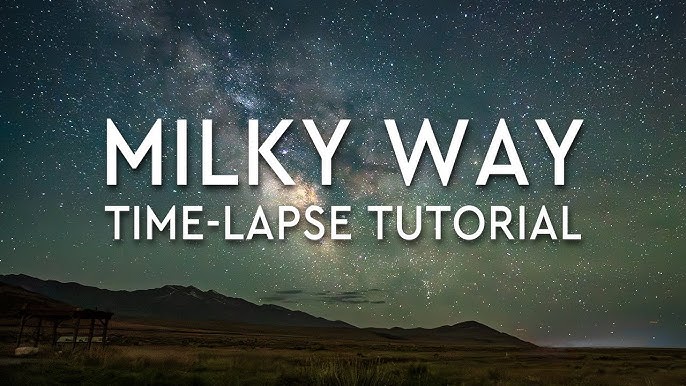This captivating image illustrates a "Milky Way Timelapse Tutorial" and showcases a stunning night sky. Dominating the scene, the Milky Way Galaxy arcs brightly above, its purplish-blue hues blending seamlessly into the darker sky, which is dotted with countless white specks of stars. Below the celestial display, the image transitions to a mountainous region, shrouded in the darkness of night, casting a silhouette against the starlit backdrop. Further down, the terrain becomes a deserted, open field, with patches of natural landscape and sparse grass. Adding a rustic element to the scene, there is a wooden frame building with open sides positioned towards the bottom left, complementing the secluded and serene atmosphere of the night. The composition is rich with color gradients, featuring whites, browns, blues, and black, enhancing the overall beauty and tranquility of this desert night setting.